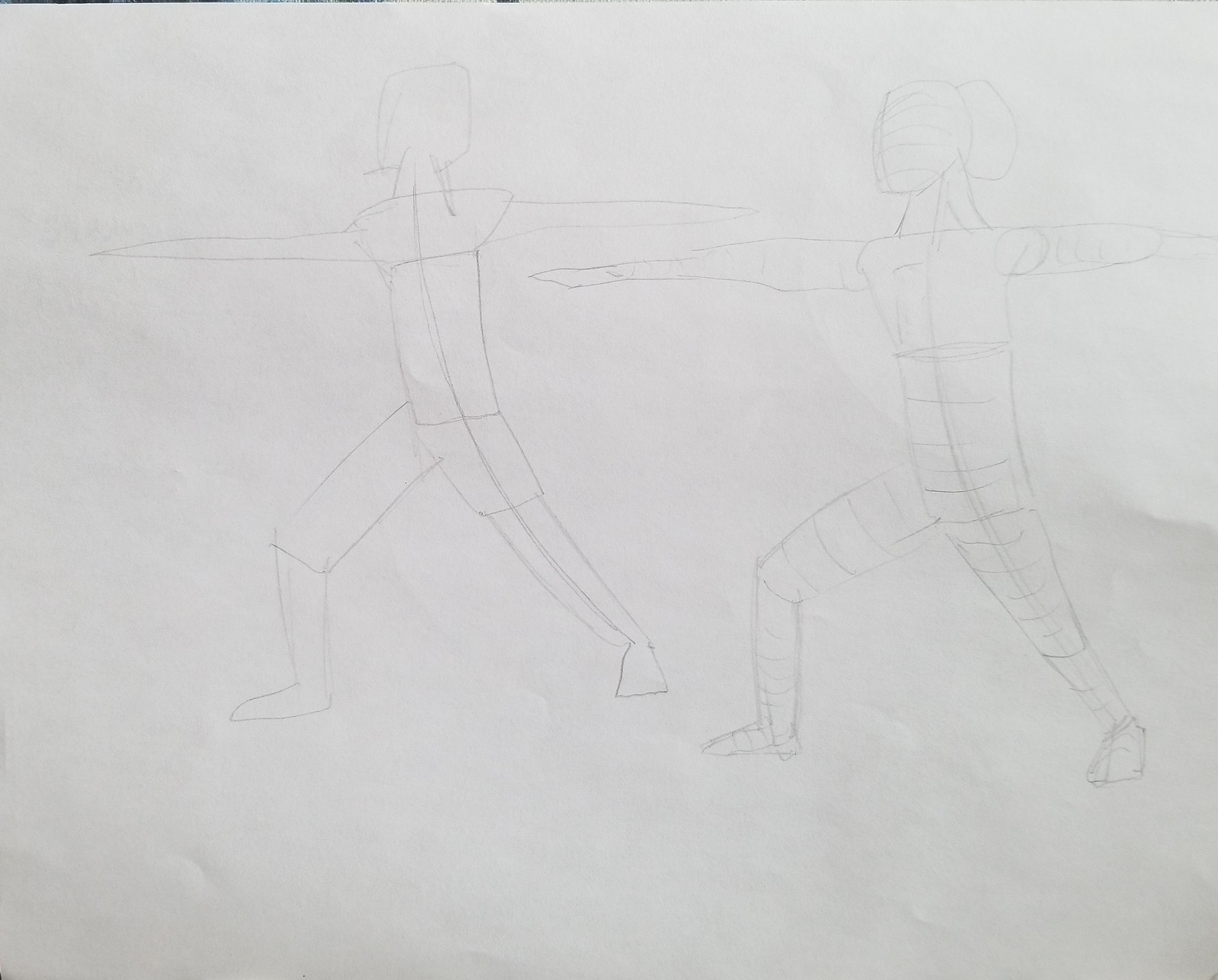This detailed black and white artwork, rendered in a square format, features two distinct figures positioned against a stark, white background. The figure on the left is depicted in a dynamic pose, with both arms extended straight out to the sides, reminiscent of a T-pose. Their right leg is placed forward, while the left leg is extended backward, offering a sense of movement or balance. The figure on the right mirrors this minimalist yet expressive style, contributing to the overall symmetry and balance of the composition. The simplicity of the black lines against the white background emphasizes the striking outline and form of the figures, creating a compelling visual story within the monochromatic palette.